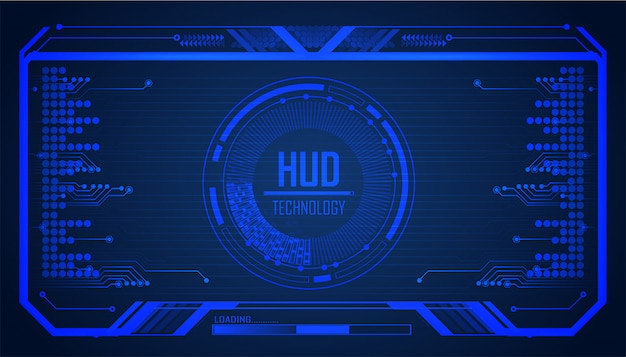The image depicts a sophisticated digital interface or HUD (Heads-Up Display) technology screen, prominently set against a black background. Central to the design is a bright blue rectangular frame, wider than it is tall, showcasing a blue-outlined circle. Inside this circle, the text "HUD Technology" is displayed, with "HUD" on top, a horizontal line beneath it, and "Technology" below the line. On both sides of the circle, multiple rows of dots are present, with some extending towards the center, suggesting connection points or data nodes. At the top of the image, a blue V-shaped graphic is featured. Additionally, a loading bar, halfway filled, spans the bottom of the screen, enhancing the look of a high-tech, game-like or computer interface environment. The overall appearance mirrors what one might see in a gaming HUD or advanced digital dashboard, providing a futuristic feel with its detailed graphical elements.